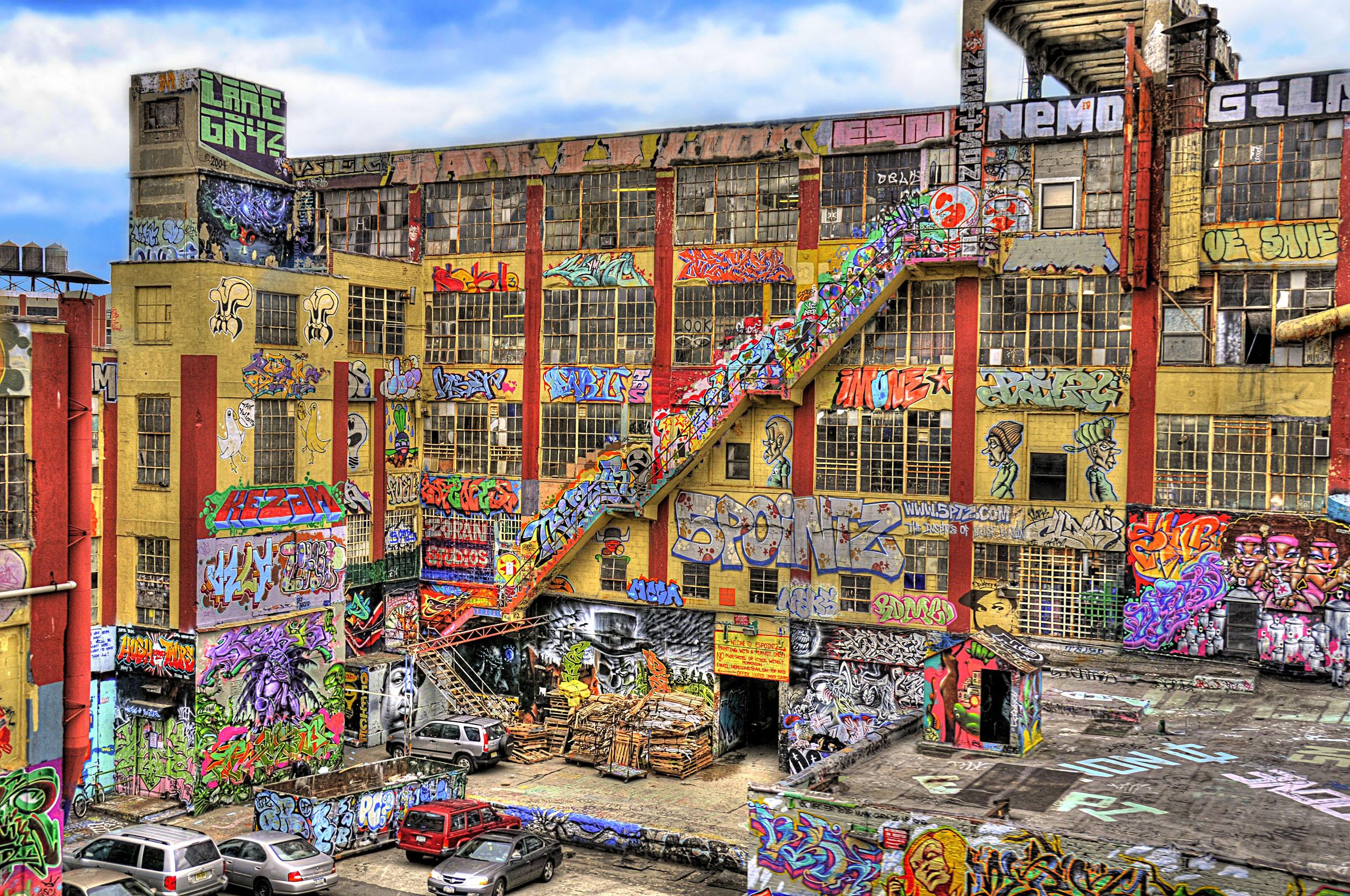This image captures the exterior of a large, yellow warehouse or factory building, heavily adorned with colorful graffiti in a riot of styles and colors, including purple, yellow, pink, and orange. Nearly every inch is covered with vibrant tags, featuring names like "Nemo," "Five Points," and "Lane Guys," as well as some drawings of faces and people. The building's facade is punctuated by numerous large and small windows, some of which are broken, adding to the urban decay aesthetic. Red bars run vertically along the structure, and a tall staircase scales its height. In the foreground, a variety of vehicles, including two gray SUVs, are parked near the building, alongside an open shipping freight container and pallets of materials. The scene is set on a cloudy daytime, underscored by a blue sky with patches of clouds.